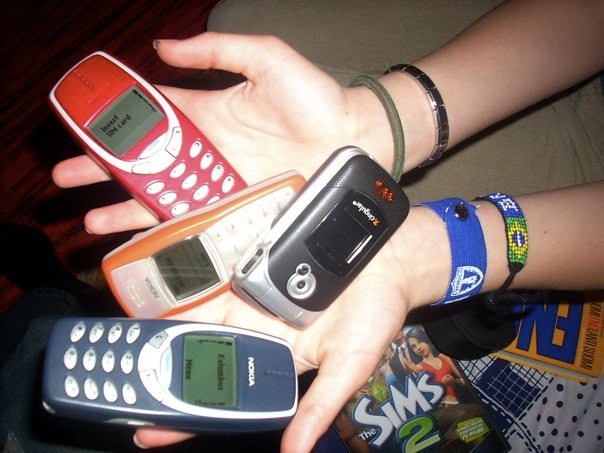This detailed photograph showcases a young Caucasian woman with light brown skin, holding four cell phones in her cupped hands, which extend from the right side of the image. Her hands and forearms bear various accessories: the upper right arm sports a green head tie and a silver bracelet/watch, while the lower arm features a blue wristband and a beaded bracelet with green, yellow, and white beads, reminiscent of the Brazilian flag.

Among the four cell phones in her hands, the topmost phone is red, below it is an orange Nokia, followed by a black and silver flip phone with a camera, and at the bottom is a blue Nokia displaying "emergency." Below her hands, a copy of The Sims 2 game lies on a bed with a yellow book featuring big blue letters, hints of smaller black and red text, and a glimpse of a reddish-brown wooden floor.